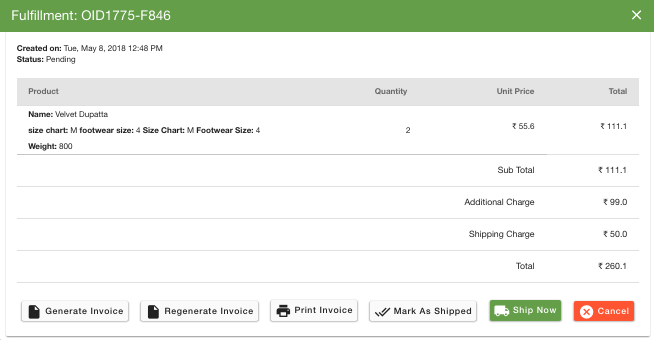In this image, set against a white background, there is a green header at the top with the white text "Fulfillment, 0ID1775F846." In the upper right corner, there is a white "X." Below the header, in bold black text, the details "Created On: Tuesday, May 8, 2018, 12:48 PM" and "Status: Pending" are displayed. A blue box is located beneath these details, divided into four columns labeled from left to right: "Product," "Quantity," "Unit Price," and "Total." Listed under the "Product" column, in white text, is the name "Velvet Dupatta." The "Size Chart" column indicates the size "M" and "Footwear Size: 4," repeated. Under these details is the "Weight: 800." Under the "Quantity" heading, the number 2 is displayed, denoting the number of items.